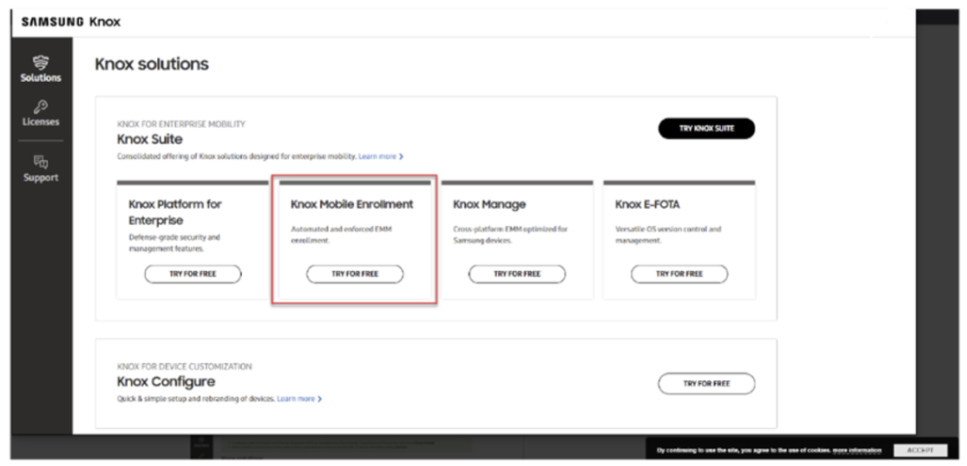The screenshot features a user interface from Samsung Knox, prominently displaying its suite of enterprise solutions. The interface consists of various sections, with "Solutions", "Licenses", and "Support" listed on the left sidebar, which has a dark gray background. The currently selected section is "Solutions", as indicated by the highlighted tab.

In the main content area, under the "Solutions" tab, we can see the heading "Knox Solutions" at the top left. Beneath this heading, there are four key options listed under "Knox Suite": "Knox Platform for Enterprise", "Knox Mobile Enrollment", "Knox Manage", and "Knox E-FOTA". Each of these options includes a button labeled "Try for Free". The "Knox Mobile Enrollment" option is notably emphasized with a red-brownish boxed outline, indicating it is selected.

Further down, there is another section for "Knox Configure", described as "Knox for Device Customization". The main display area is set against a white background, contrasting with the dark gray sidebar. Despite some text being blurry, the central features of the interface and the structure of the navigation are clearly identifiable.